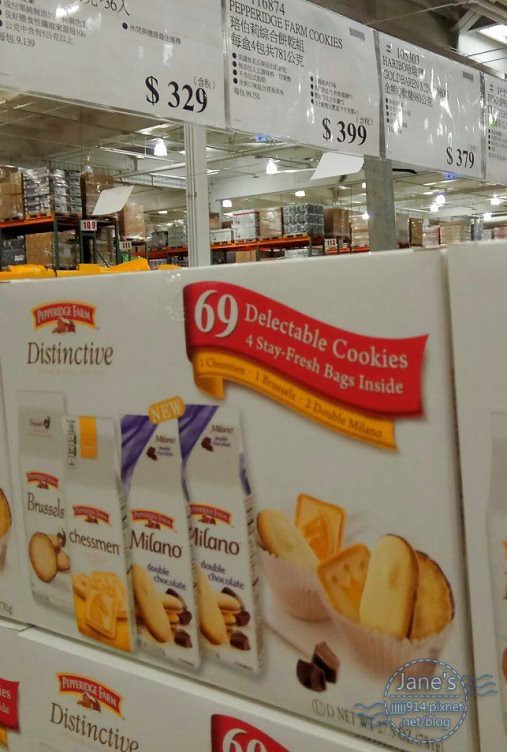This image captures a bustling scene inside a large wholesale grocery store, resembling a Costco environment, possibly located outside the United States, perhaps in a Chinatown area. Dominating the foreground is an eye-catching advertisement for Pepperidge Farm cookies, highlighting an assortment of 69 delectable treats neatly divided into four stay-fresh bags. The packaging prominently displays pictures of the different cookie varieties, including Milanos, Chessmen, and possibly Bruschetta, though the exact details are somewhat hard to discern. The advertisement features a red banner emphasizing the "69 delectable cookies," adding a splash of color to the scene.

In the background, large white signs with black text indicate product prices and details, contributing to the warehouse ambiance. These signs are set against towering shelves stocked with a myriad of products, reminiscent of Costco's bulk-buying layout. The overhead ceiling, adorned with industrial lighting, completes the expansive and well-illuminated shopping environment. This vibrant and detailed setting, coupled with the colorful cookie images, suggests an era that feels contemporary yet universally familiar.